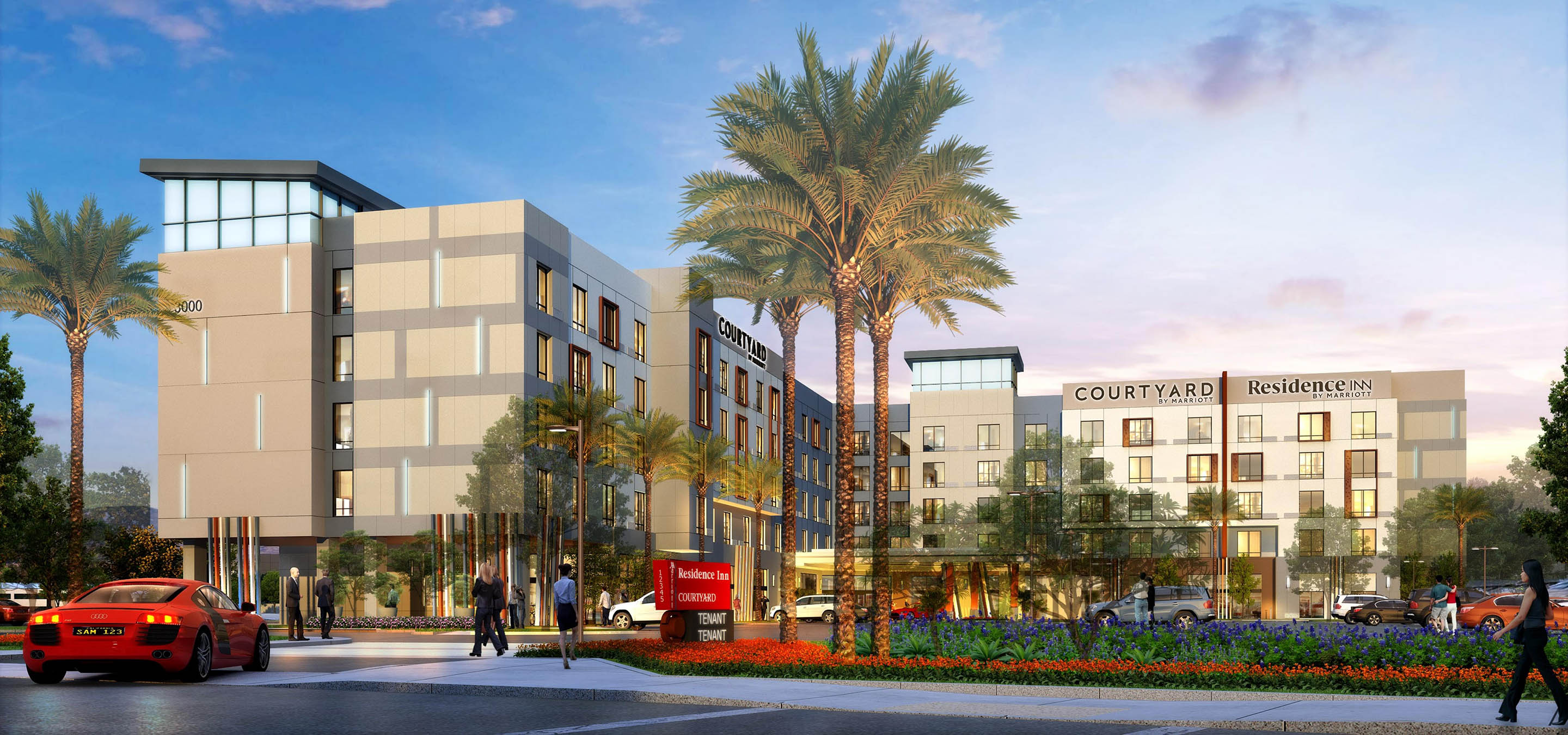The computer-rendered image depicts a large, L-shaped Courtyard Residence Inn hotel, standing at about four to five stories high. The structure is primarily gray with numerous windows and dark gray roofs, typical of a hotel. The setting suggests a warm climate, possibly Miami, indicated by the presence of several palm trees in the foreground. 

On the left side of the image, a striking red, mid-engine Audi sports car (license plate SAN123) is prominently visible, heading towards the hotel entrance. Surrounding the entrance area, there is a well-maintained landscape featuring a bushel of orange flowers with purple ones behind them, and a red sign with some unreadable text. 

In front of the hotel, various pedestrians can be seen, including a woman walking on the sidewalk. The scene captures a sunny, vibrant day with lots of activity, creating a welcoming atmosphere around the Courtyard Residence Inn.